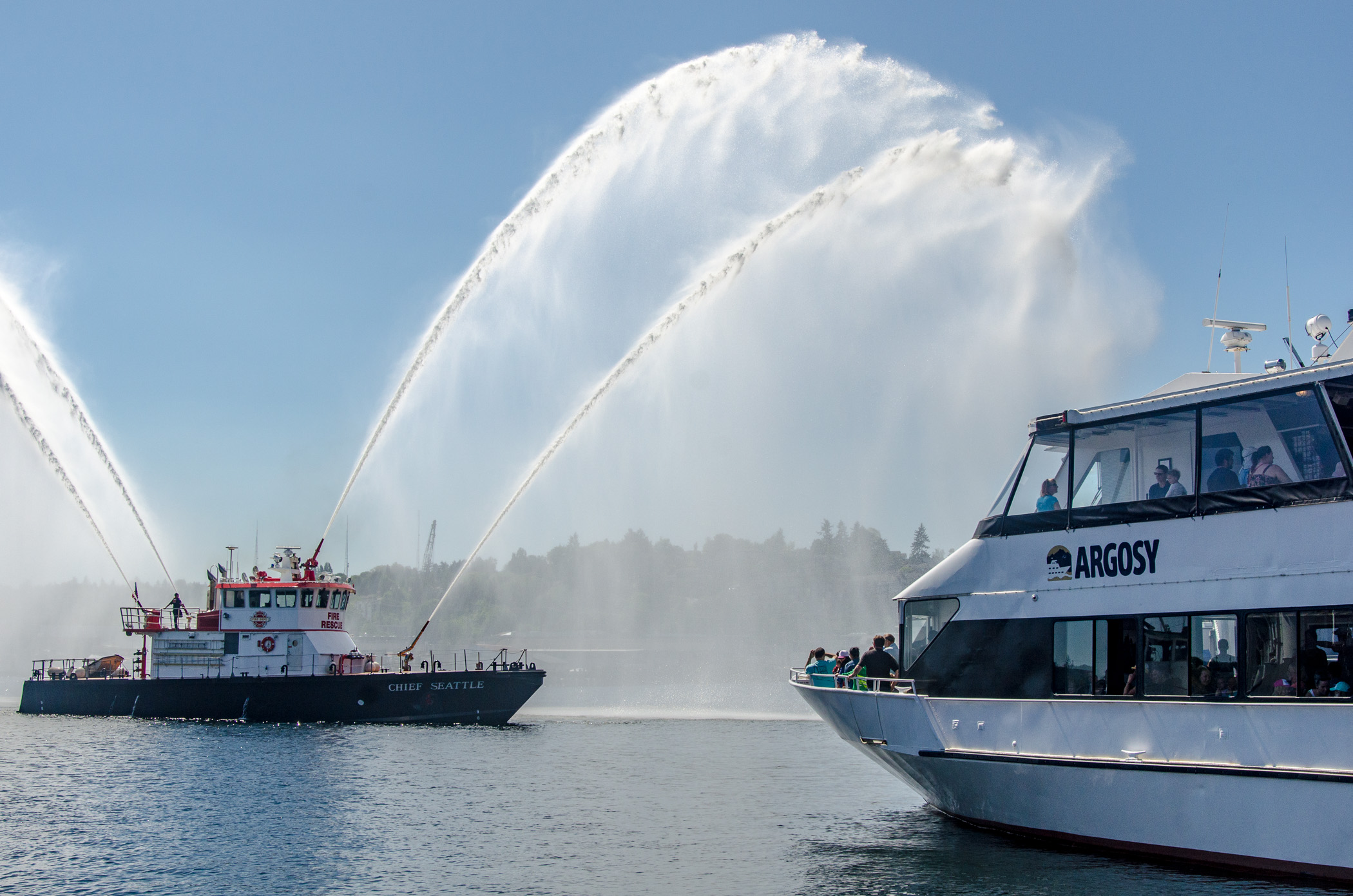In this image, we see a serene lakeside scene under a clear blue sky. Dominating the foreground, a vibrant fireboat, approximately 30 to 40 feet long, commands attention as it sprays water from four powerful jets, sending streams nearly 100 feet into the air. The fireboat features a blue hull with "Chief Seattle" inscribed in white on its side, and its upper structure is stark white. At the top, middle, and back of the boat, the water jets create misty clouds that blend with the tranquil backdrop.

Positioned to the right side of the image is a two-level tour boat filled with onlookers. This boat, painted white with a black lining and prominently displaying the name "Argosy," functions much like a ferry. The decks are enclosed, providing comfort to its passengers as they observe the scene and the spectacle of the fireboat. The tour boat is situated in the lower right corner, moving towards the middle right of the frame.

The entire scene is set against a calm lake with a lush forest and possibly a couple of cranes visible in the background, enhancing the natural beauty of this outdoor daytime setting. The image captures an interplay of colors, including whites, blacks, grays, various shades of blue, and hints of red, adding to the vividness of the moment.